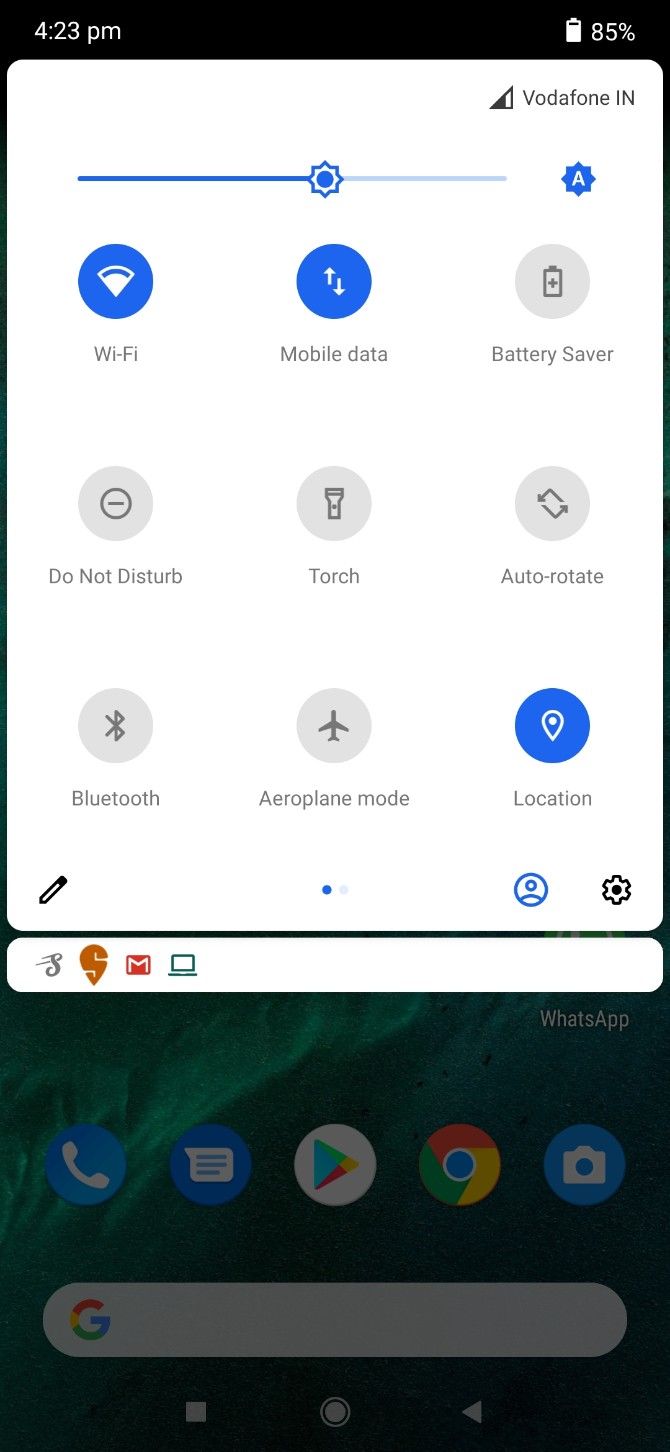A screen capture of a cell phone display shows it is 4:23 p.m. with the battery at 85% charge. The device is connected to the Vodafone IN network, indicating a possible location in India. The quick settings panel is open, revealing several toggles including Wi-Fi, mobile data, battery saver, Do Not Disturb, torch, auto-rotate, Bluetooth, airplane mode, and location. Of these, Wi-Fi, mobile data, and location are activated and highlighted in blue, while the others remain gray. The brightness slider indicates the brightness is set to just above the halfway mark. Below the settings panel, the home screen is partially visible, featuring a WhatsApp shortcut and a Google search bar at the bottom. Additional visible app icons are for Phone, Messaging, Google Play Store, Google Chrome, and Camera.